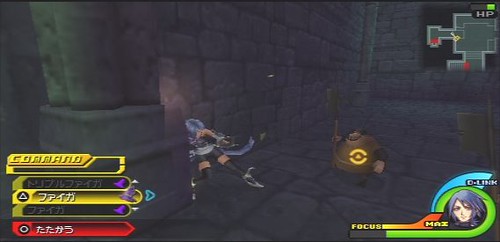This landscape-oriented screenshot from a video game, approximately three and a half times as wide as it is tall, depicts an action-adventure scene set in a dimly lit dungeon or castle with large, thick stone walls and stone floors. At the center, a small female fighter with long, grayish-purple hair stands poised for battle. She sports sleeveless armor, black shorts, and long leggings that leave her thighs visible. Her face is turned away, and she wields a sword in her right hand and an indeterminate weapon in her left. To her right stands a squat, circular robot with a beige color, marked with a bright oval featuring a semi-circle on both the top and bottom, plus a filled circle in the middle. 

The lower left corner displays game stats, with yellow and red text including the word "command" and a triangle symbol, possibly accompanied by Asian characters. The lower right corner shows an icon of the female character with text reading "D-Link" and "Mei," along with metrics like "focus" and "max," indicative of her health or energy. A map in the top right corner, labeled "HP," likely tracks their location or mission progress. The dark, old-school aesthetic of the setting conveys a Minecraft-like environment constructed of large rock bricks, enhancing the medieval atmosphere of the scene.